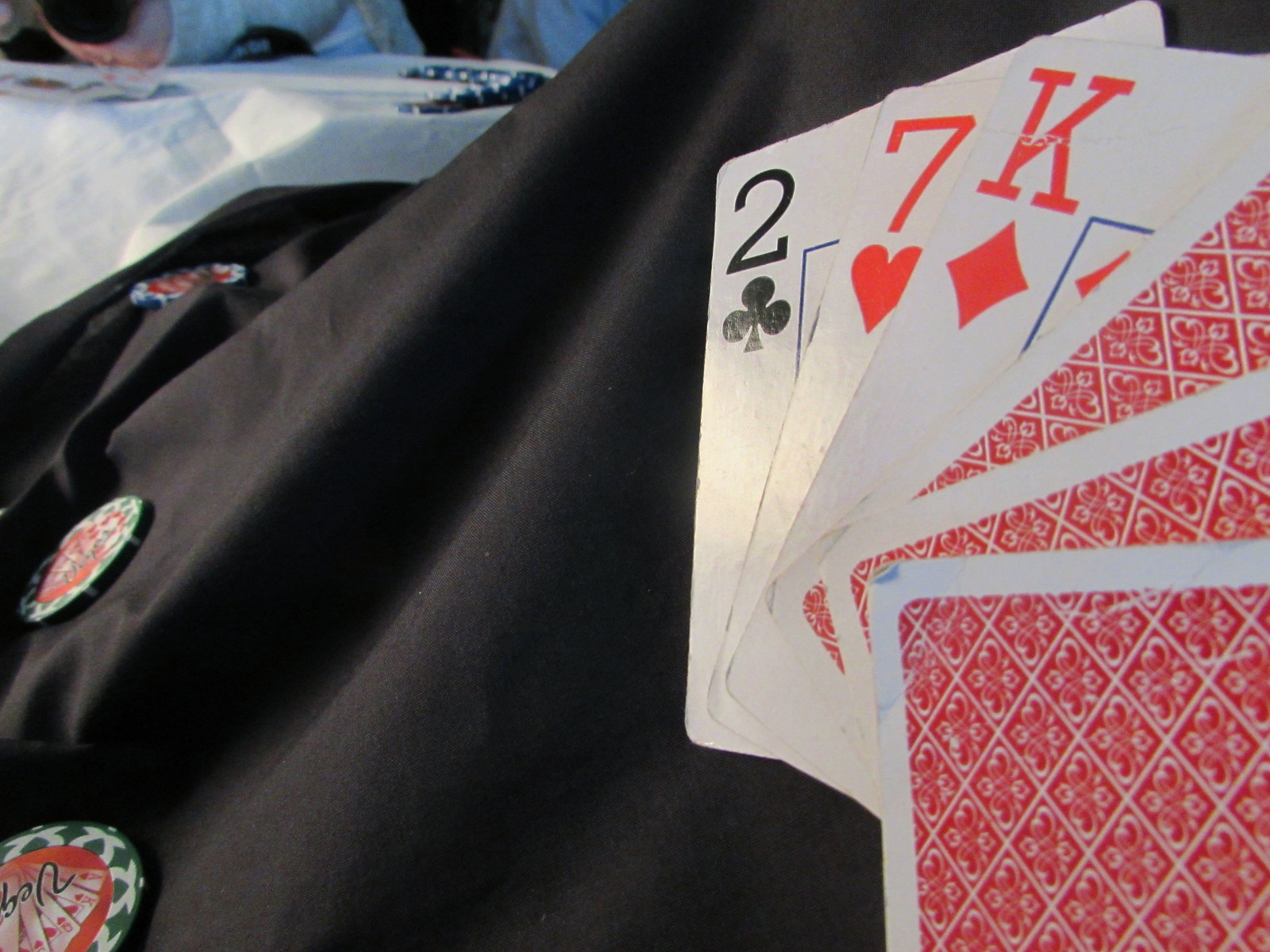The image features an intimate, close-up photograph of six playing cards arranged on a wrinkled black tablecloth. The three cards at the forefront are visible and identifiable: the Two of Clubs, the Seven of Hearts, and the King of Diamonds, each slightly overlapping the one beneath it. The remaining three cards, also overlapping in a similar manner, are face-down, showcasing a red pattern with white borders on their backs.

Resting on the same black tablecloth to the left, there are three poker chips: two with green, red, and white coloration, and one with blue, red, and white accents. The background of the image is intentionally blurred but reveals a white table covered by a white tablecloth, with several blue poker chips scattered atop. The photograph’s primary focus remains sharply on the trio of face-up cards, emphasizing their prominence amidst the subtle surroundings.